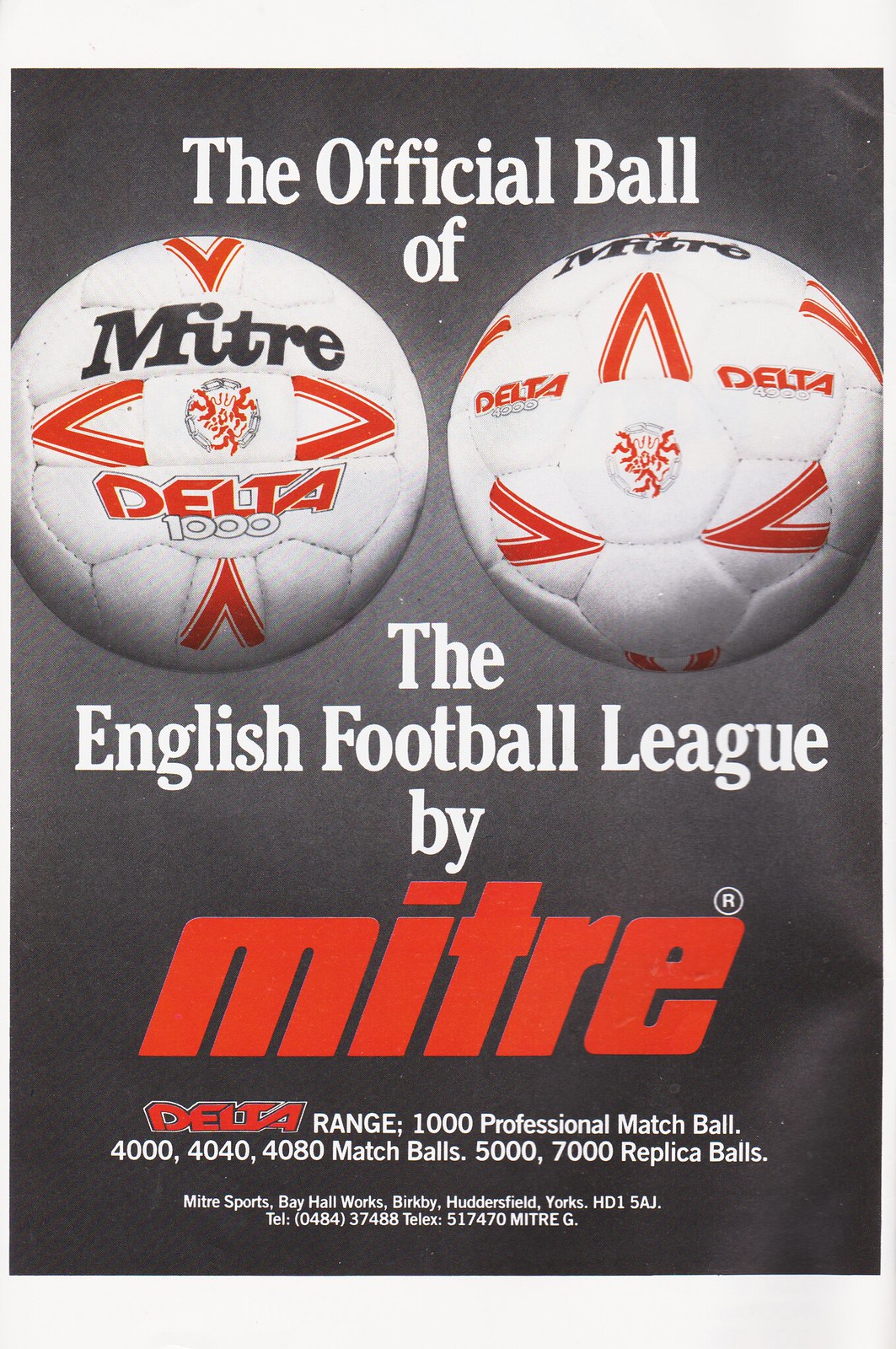This image is an advertisement for Metri soccer balls, featured in a grayscale photograph that appears to be from a magazine or sports program. Dominating the top half of the ad, two soccer balls are prominently displayed side by side, showcasing their red, white, and black design. The brand name "METRI" is clearly printed in black letters on one of the balls, accompanied by an arrow design and the model name "Delta 1000" in white letters. The ad emphasizes that this is the official ball of the English Football League, a detail which is reiterated above and below the ball. At the bottom of the ad, contact information, including an address in Hattersfield, New York, and a phone number, is provided. The ad highlights Metri's offering of various categories of replica balls, inviting potential customers to explore their range.